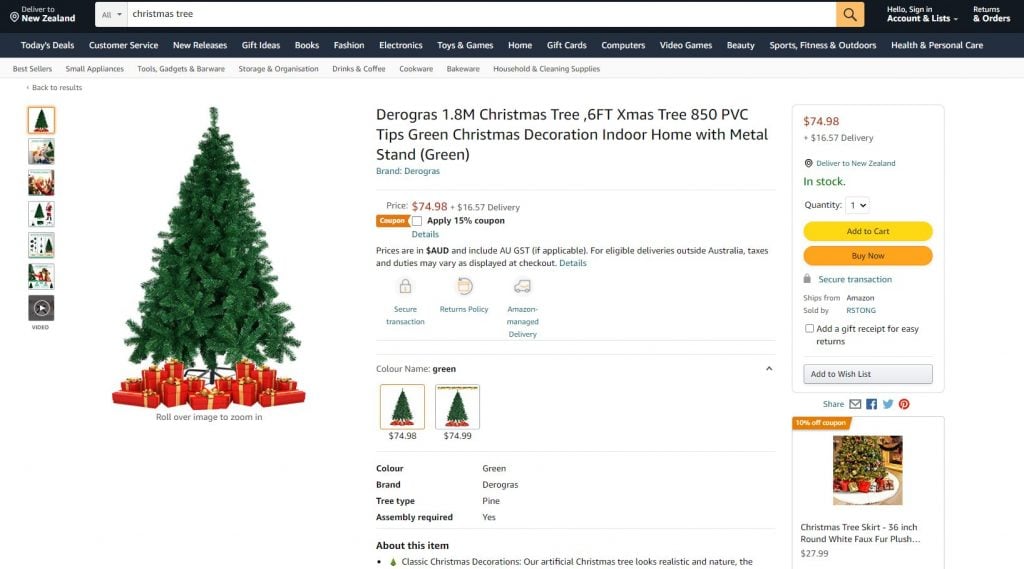This image captures a detailed screenshot of an Amazon ordering page viewed on a desktop or laptop computer. The user has notably searched for a Christmas tree, as indicated by the tangible keyword in the search bar. The prominent feature of the page is an image displaying a well-decorated Christmas tree with numerous gifts underneath. The search appears to be conducted from New Zealand, as marked by the regional settings in the top left corner of the screenshot. 

Additionally, the user is not signed into an Amazon account. The top taskbar provides various shopping categories available for exploration. The specific product under consideration is a "Darrow Grass 1.8M Christmas Tree," which is described in detail as a six-foot tall tree featuring 850 PVC tips and designed for indoor use. It comes with a green metal stand, and is currently priced at $74.98, supplemented by a $16.57 delivery charge. A 15% discount coupon is also available for this item.